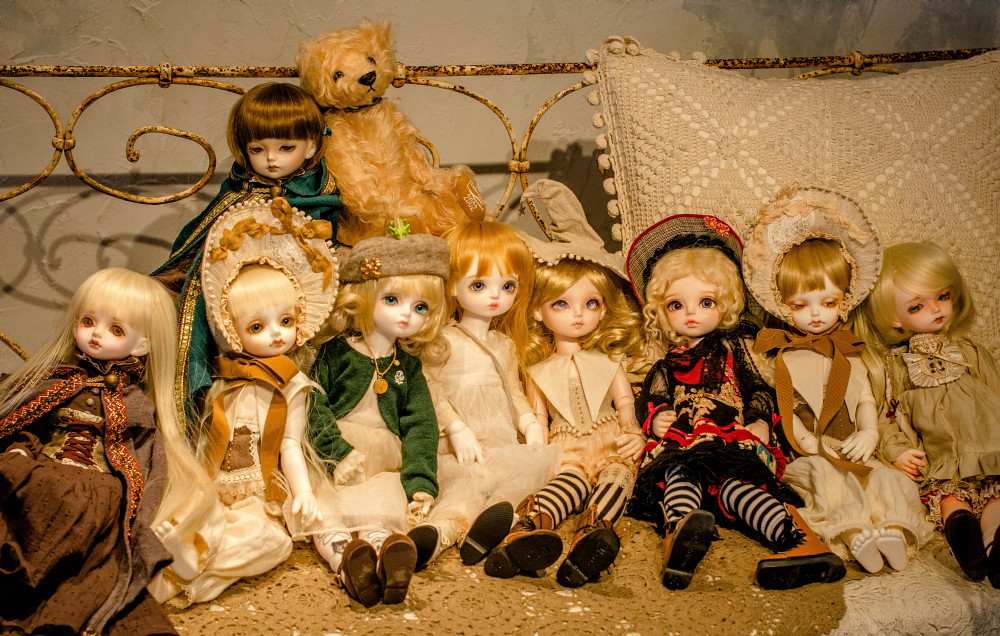In this vintage-style photograph, nine intricately dressed Asian ball-jointed resin dolls and one lanky tan teddy bear are meticulously arranged on an aged white, rusted cast iron day bed against a white wall. The dolls, with their striking pale complexions, small mouths, and large glass eyes, exude a neutral serenity. They are adorned in an array of gothic Lolita costumes, predominantly in earth tones with accents of red and black, channeling an elegant Victorian aesthetic. The bed is draped with crocheted tan doilies, enhancing the antique ambiance. Positioned in two neat rows, eight blonde dolls sit below, with the fourth doll from the left showcasing a unique strawberry blonde hue. Above them sits a distinct doll with short brown hair, next to the teddy bear characterized by beady black eyes and nose. A large cream cushion rests on the right, providing a backdrop for three of the dolls to lean against. The overall scene combines modern elements with a deliberate vintage charm, reflected in the detailed styling and rustic setting.